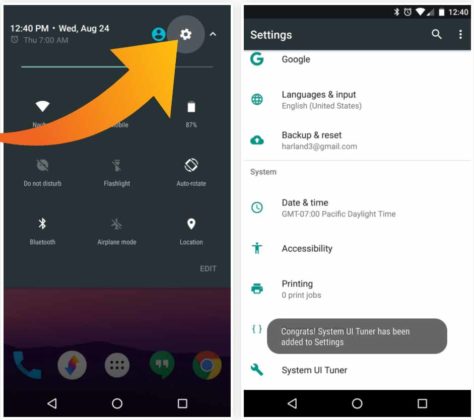This screenshot displays the home page of a smartphone, specifically showcasing the settings menu. At the top of the screen, there's a prominent orange ombre gradient arrow pointing towards the settings icon, which resembles a gear wheel. This visual cue directs the user to explore the settings functionality. Upon clicking the settings icon, the user is presented with a comprehensive list of options, including Google, Languages & Input, Backup & Reset, System, Date & Time, Sound, Accessibility, and Printing (noting there are zero print jobs). Additionally, there's a congratulatory message indicating that the System UI Tuner has been successfully added to the settings menu. The System UI Tuner is designed to allow users, particularly those who may not be very technology-savvy, to customize and optimize their phone's interface, ensuring the device operates at peak performance. This feature helps manage the system's design and functionality in the background, assisting in maintaining the overall user experience.